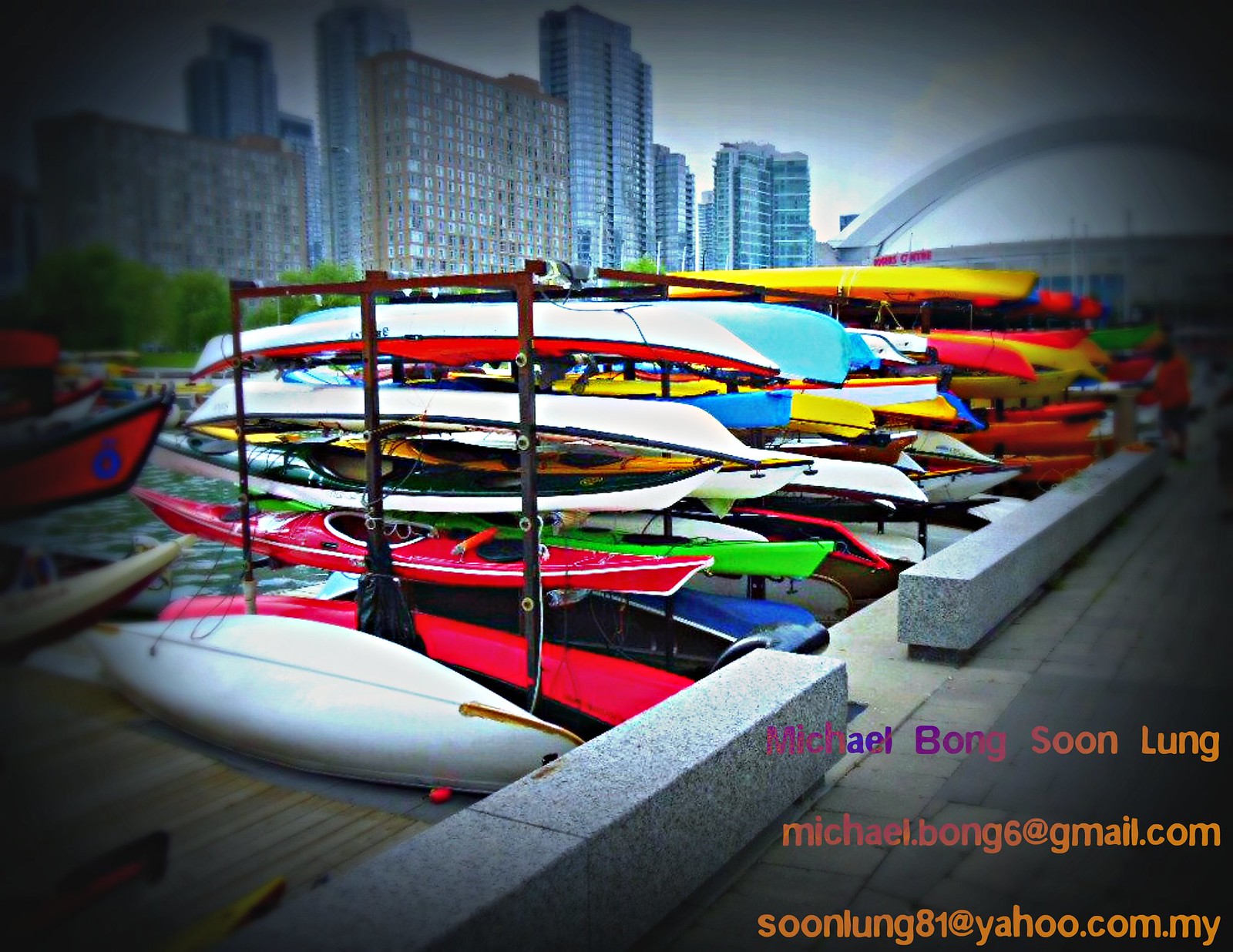The landscape-oriented, color photograph showcases an extensive collection of vibrant kayaks neatly stacked in rows, five or six high, along a quay in an urban setting. The kayaks, awash in hues of hot pink, yellow, blue, white, and their combinations, are situated to the left of a pedestrianized walkway, which features two gray flat benches. The bottom right of the image includes the contact details: "MichaelBongSoonLung," "Michael.Bong6 at gmail.com," and "SoonLung81 at yahoo.com.my," in a mix of purple, blue, pink, yellow, and orangish-yellow text. In the background, a serene body of water shimmers, accompanied by hints of boats sailing. Towering above are skyscrapers in shades of blue and brown, punctuated by patches of greenery, completing the picturesque urban waterfront scene.